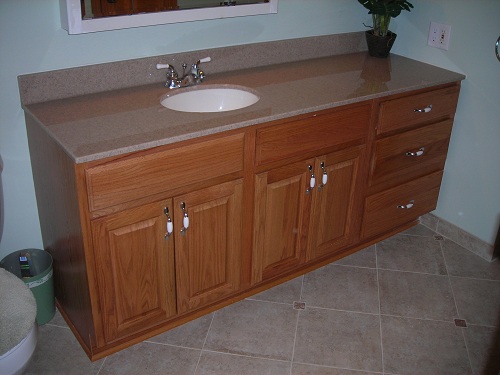A dimly lit bathroom showcases a sophisticated vanity set against a baby blue painted wall. The vanity features a single sink with ample counter space and appears designed to potentially accommodate a second sink. Its cabinetry is crafted from a wood slightly darker than oak, possibly cherry wood, and is adorned with decorative silver metal and white pearl handles. The arrangement includes three drawers and two double-faced cabinet doors. An artificial plant in a pot occupies the counter's corner, adding a touch of greenery. A mirror is mounted above the vanity, and a light switch, possibly equipped with a dimmer, is visible on the right-hand side of the wall.